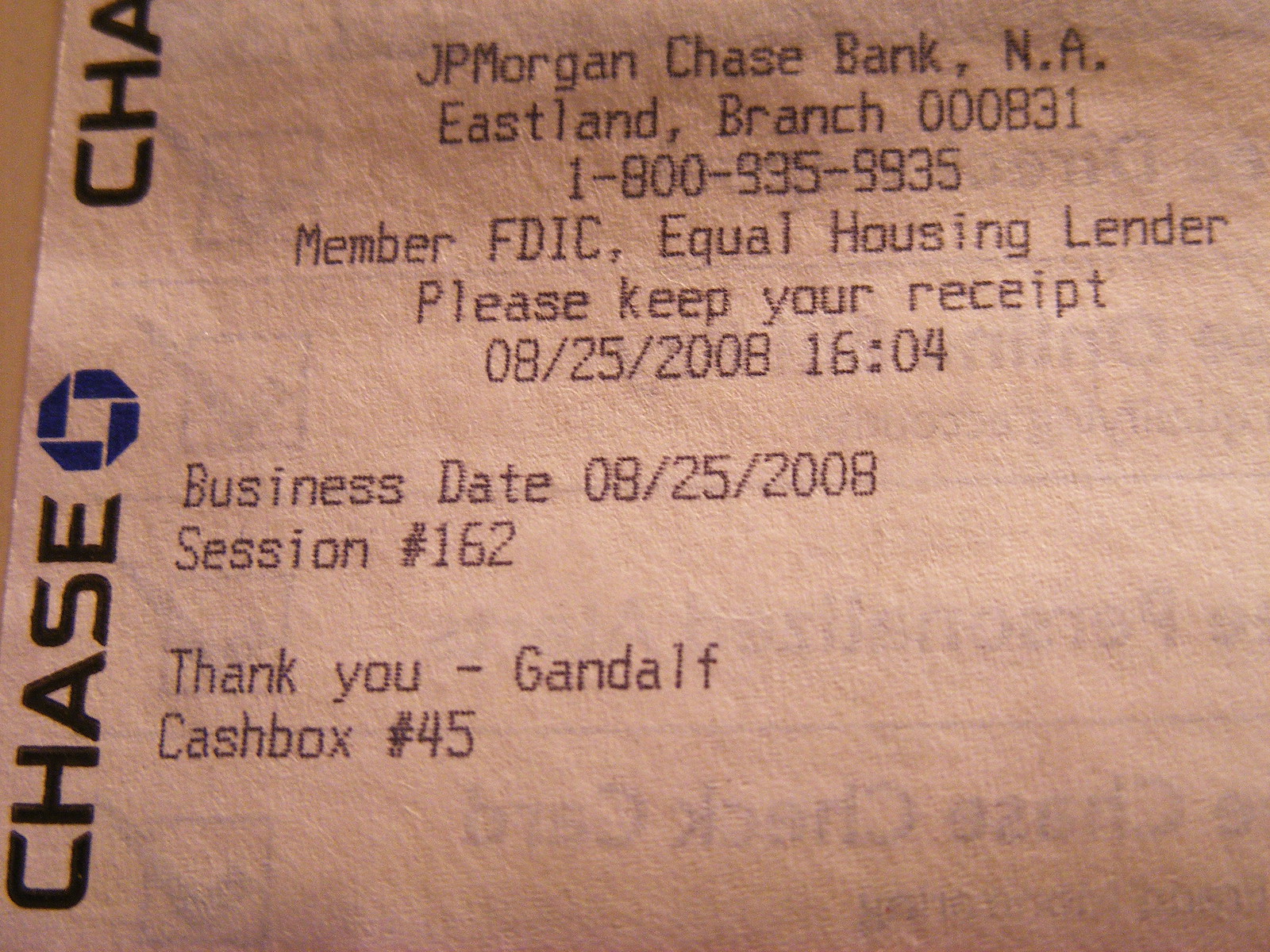Here is a detailed and cleaned-up caption for the image described:

---

A detailed receipt from JPMorgan Chase Bank's Eastland branch, with the zip code 000831. This official document, dated August 25, 2008, at 4:04 PM (session 162), records a transaction conducted by sales associate Gandalf. The transaction possibly pertained to safe deposit box number 45. The receipt features all-black text and a vertical "Chase Bank" label on the left, accompanied by the iconic blue Chase Bank symbol. The bank is identified as a member of the FDIC and an Equal Housing Lender.

---